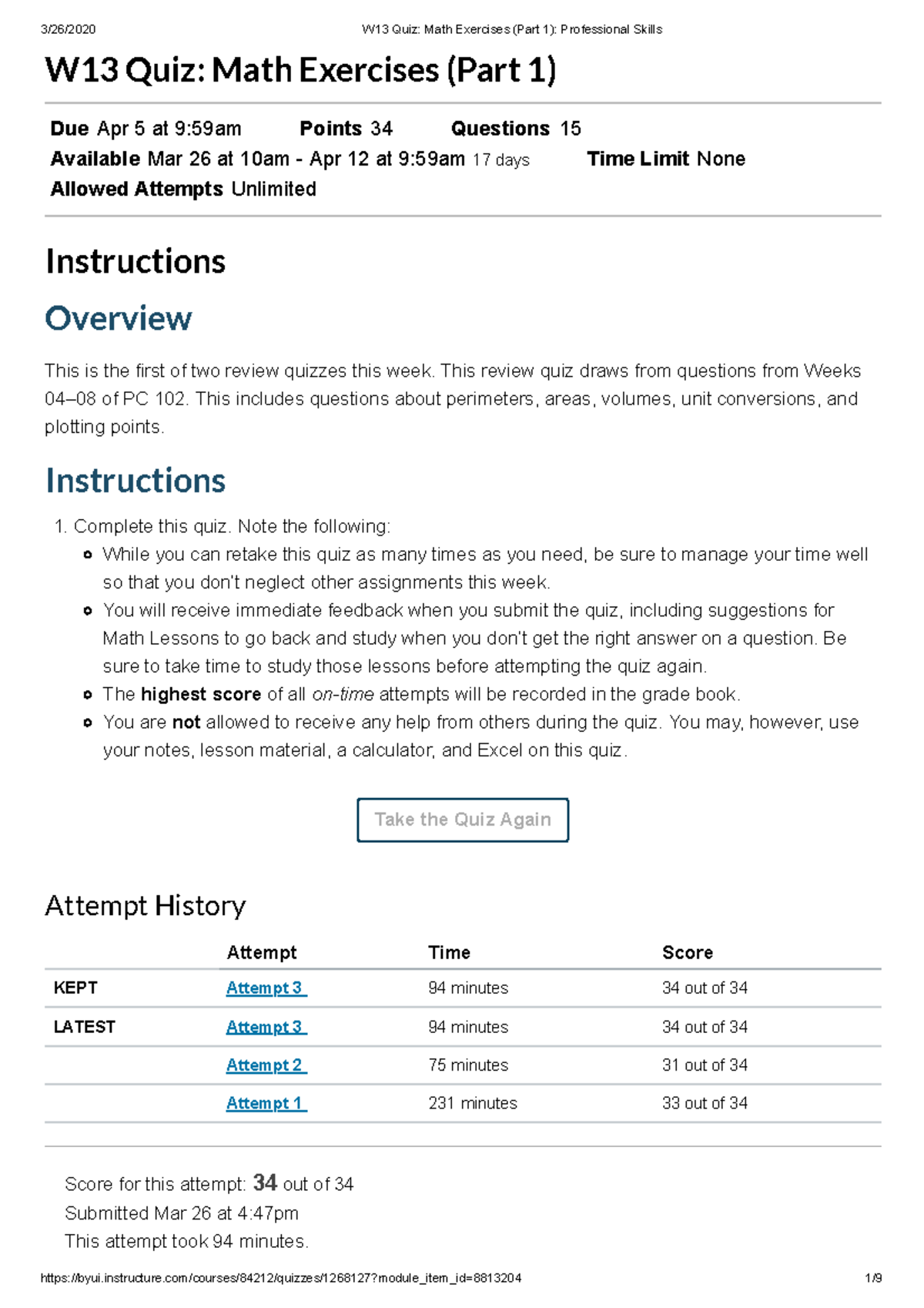Here is the detailed and cleaned-up caption for the image:

---

The image prominently displays a quiz overview and instructions on a clean white background, featuring both black and blue text. 

At the very top, the header reads "W13 Quiz: Math Exercises - Part One, Professional Skills." In the upper-left corner, key information is noted: 
- Date: 3/26/2020
- Due Date: April 5th at 9:59 a.m.
- Points: 34
- Questions: 15
- Available: March 26th at 10 a.m. through April 12th at 9:59 a.m. (17 days)
- Time Limit: None
- Allowed Attempts: Unlimited

Below this, there are sections for "Instructions" and "Overview." 

The overview explains that this is the first of two review quizzes for the week, covering content from weeks four through eight of PC 102. It includes topics such as parameters, areas, volumes, unit conversions, and plotting points.

The instructions specify the following:
- You can retake the quiz multiple times, but manage your time wisely to avoid neglecting other assignments.
- Immediate feedback is given upon submission, including suggestions for math lessons to revisit when answers are incorrect.
- The highest score from all attempts will be recorded in the gradebook.
- No help from others is allowed, but you may use notes, lesson materials, a calculator, and Excel.

A button labeled "Take the Quiz Again" is visible, along with an "Attempt History" section. The history lists three attempts:
- Attempt 1: 94 minutes, score 34/34
- Attempt 2: 94 minutes, score 34/34
- Attempt 3: 75 minutes, score 31/34

Another line shows a summary of the current attempt:
- Score: 34/34
- Submitted on: March 26th at 4:47 p.m.
- Time taken: 94 minutes